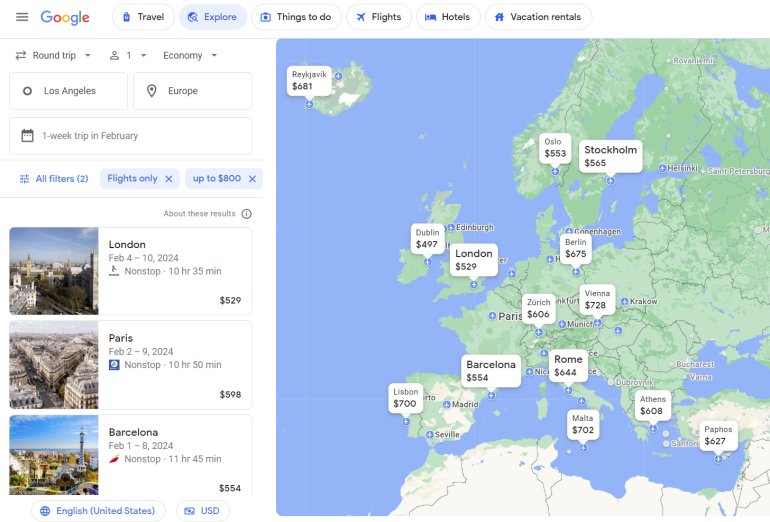The screenshot is of Google search results, specifically within the "Explore" tab of a travel search interface. In the top left corner, the Google logo is visible. Below the logo, there are several navigation buttons such as "Travel," "Explore" (which is highlighted in a faint blue, indicating the active tab), "Things to Do," "Flights," "Hotels," and "Vacation Rentals."

On the left side of the interface, there are various travel filters and preferences. The settings indicate a "Roundtrip" with one traveler (denoted by a person icon with the number 1) in economy class. The search query specifies travel from Los Angeles to Europe for a one-week trip in February.

On the right side, a digital map displays several European cities marked with price indicators for flights. For example, Berlin shows a price of $175, Athens appears to be $608, and Rome is listed at $644.